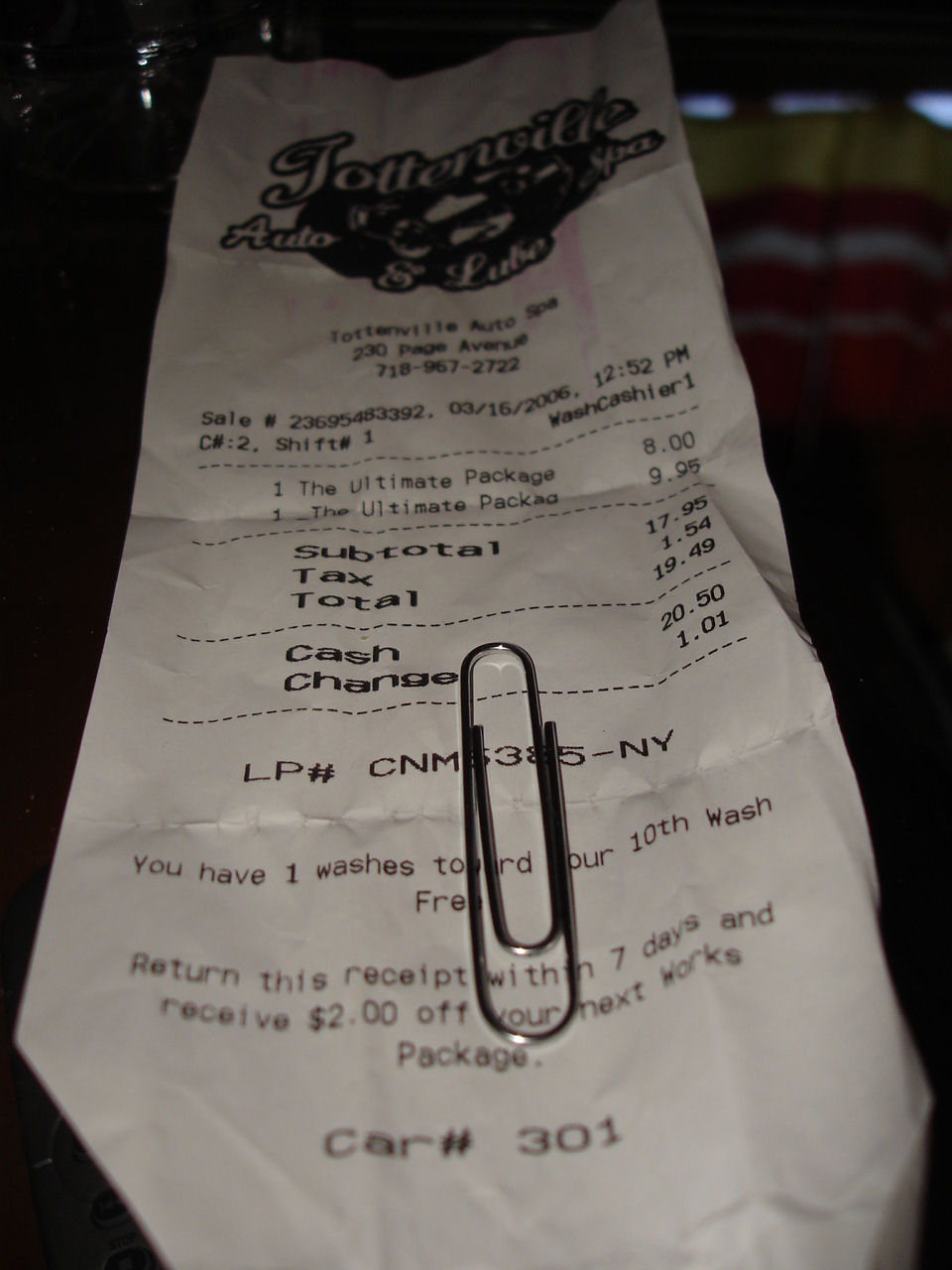This is a detailed close-up, color photograph in portrait format showcasing a crinkled, white receipt from Tottenville Auto Spa and Lube, located at 230 Page Avenue, with a phone number of 718-267-2722. The receipt reveals a purchase made on March 16, 2006, at 12:52 PM, including two Ultimate Packages, oddly priced at $8.00 and $9.95 respectively. The subtotal amounts to $17.95, with an additional tax of $1.54 bringing the final total to $19.49. The image captures a paperclip resting in the middle of the receipt, which is lying on a glossy wooden surface, hinted to be a bar top, as evident by the blurry wine or cocktail glasses visible in the background. The payment method was a $20.50 cash transaction, resulting in a change of $1.01. The car serviced is noted as car number 301. The overall composition places emphasis on the detailed transaction record while subtly indicating the surrounding setting.